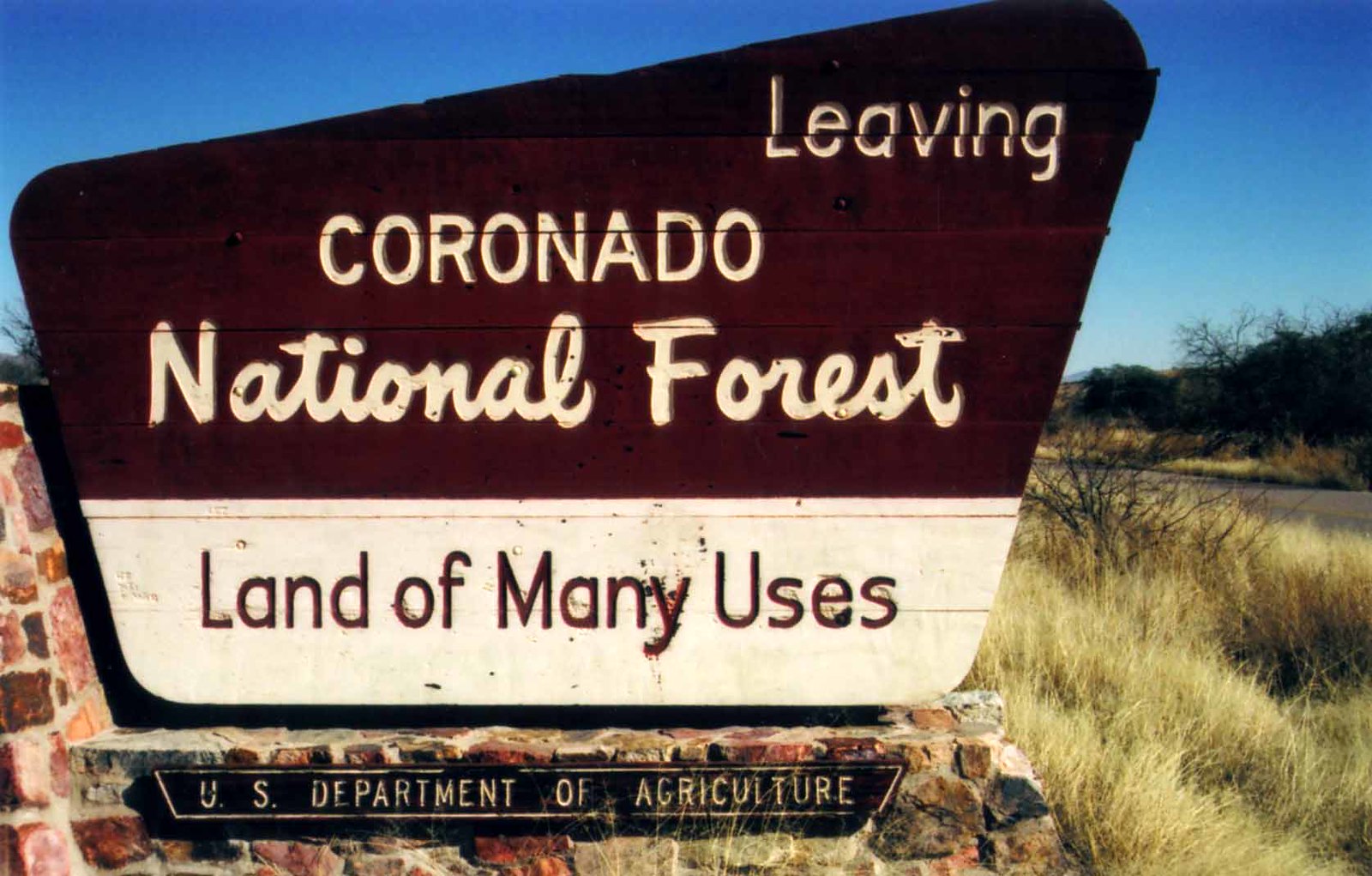This outdoor image captures a large road sign mounted on a multi-colored stone platform, which includes shades of black, brown, and red. The sign prominently features a red top section that slants upwards to the right, with white text reading "Leaving Coronado National Forest." Below this, the lower, white section of the sign states "Land of Many Uses" in red print. A small plaque at the base of the sign reads "U.S. Department of Agriculture." The platform itself is constructed from an array of bricks that rise on the left side of the sign and descend towards the right. In the foreground to the right, there is a ditch area with tall, brownish-yellow grass and a leafless shrub, indicating a dry season. Beyond this, a road stretches across the image, with more brush and grass visible on the far side. The background showcases a clear blue sky, adding a serene touch to the landscape.